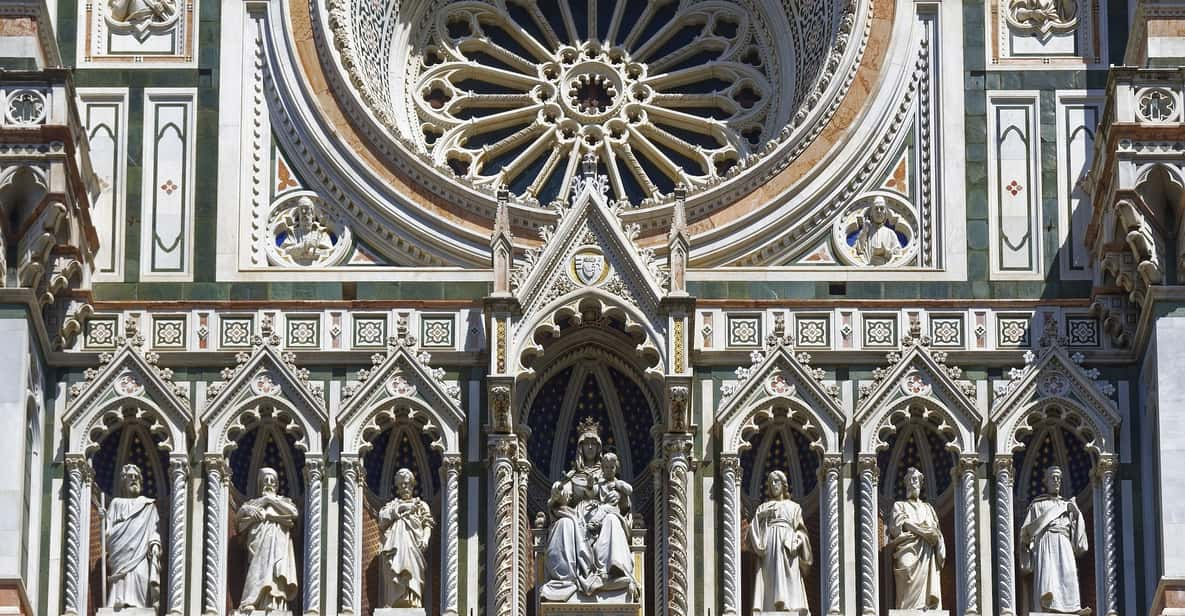This photograph captures the intricate middle portion of a heritage building or tourist spot with sophisticated, royal architectural design, possibly resembling a structure like Notre Dame. Sunlight bathes the scene, highlighting a central, large circular motif at the top, resembling a flower made from cream and brown colors. Surrounding this key feature are sculptures of human figures crafted from cream-colored materials. The middle section of the photo showcases detailed carvings and dark green tiled patterns. Lower down, there are more designs and statues, including a prominent entrance with an arch and triangular rooftop characteristic of medieval Gothic churches. The structure, likely made of marble, exudes symmetry and meticulous craftsmanship that seamlessly blend varied curves, patterns, and sculptures.